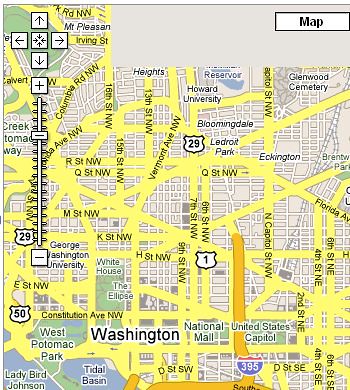This is a detailed, color image of an older-style map, reminiscent of MapQuest, showing the Washington, D.C. area. The map highlights the region's roadways primarily with yellow lines crisscrossing in various directions. Notable routes include highways such as Highway 29, Highway 1, Highway 50, and Interstate 395, with smaller neighborhood streets depicted by white lines. Key landmarks labeled include the U.S. Capitol, National Mall, White House, West Potomac Park, Tidal Basin, The Ellipse, and prominent institutions like George Washington University and Howard University. Additional areas noted are Glenwood Cemetery, Bloomingdale, LeDroit Park, Ekington, with streets like Columbia Road NW, Irving St, 16th St NW, M St NW, K St NW, and H St NW. The map interface features navigational arrows on the upper left, a "map" icon in the upper right, and zoom controls to adjust the view.